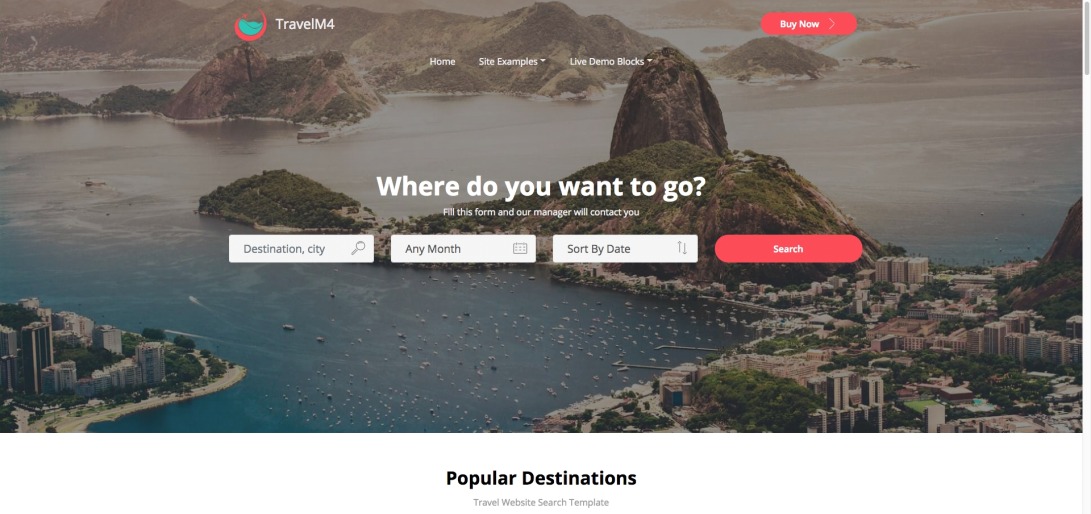This screenshot captures the homepage of the TravelM4 website, showcasing its clean and user-friendly interface. 

In the top-left corner, the website's logo "TravelM4" is prominently displayed, while the top-right corner features a conspicuous "BuyNow" button. Directly below these elements in the center of the page, several navigation options are listed horizontally in white text, including "Home", "Site Examples", and "Live Demo Blocks".

Dominating the middle of the screen is a large, bold text asking, "Where do you want to go?" Below this, a smaller text prompts visitors with, "Fill this form and our manager will contact you."

The central section of the webpage features four primary interactive elements:
1. A search box labeled "Destination City" with an accompanying magnifying glass icon.
2. A date picker labeled "Any Month" featuring a small calendar icon.
3. A sorting option labeled "Sort by Date" with up and down arrows to adjust the sorting order.
4. On the far right, a large red button with white text labeled "Search" invites users to begin their travel search.

The background image of the website sets a relaxing tone with a picturesque view of a city located adjacent to clear blue waters, giving off a tropical vibe.